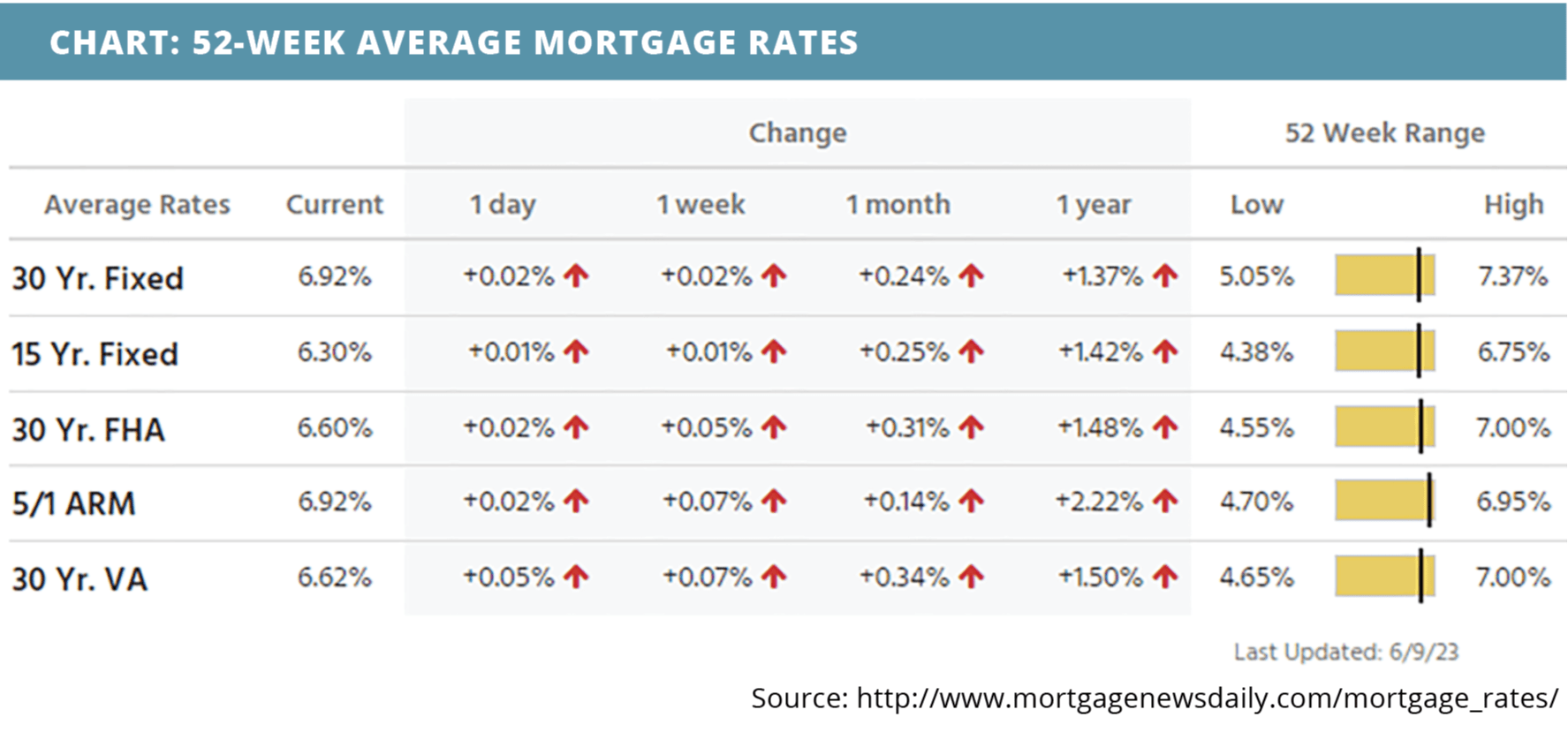Screenshot Description:

The screenshot features a header bar in turquoise blue with bold, white, all-capitalized text that reads "CHART: 52-WEEK AVERAGE MORTGAGE RATES." Below the header, columns titled "Average Rates," "Current," "1 Day," "1 Week," "1 Month," "1 Year," "Low," and "High" extend horizontally across the image. 

Vertically aligned on the left side are different types of mortgage loans, listed as "30 Year Fixed," "15 Year Fixed," "30 Year FHA," "5/1 ARM," and "30 Year VA." Each loan type is associated with a series of boxes filling in the respective values for the periods indicated in the top columns. 

The screenshot details these mortgage rates, showcasing fluctuations and averages over various time frames. For instance, the current rate for a "30 Year Fixed" mortgage is shown at 6.92%. At the bottom of the screenshot, the source of the data is indicated by a website URL. 

Overall, this detailed chart provides an organized view of average mortgage rates over different timescales, giving readers a clear visual of how rates have varied.